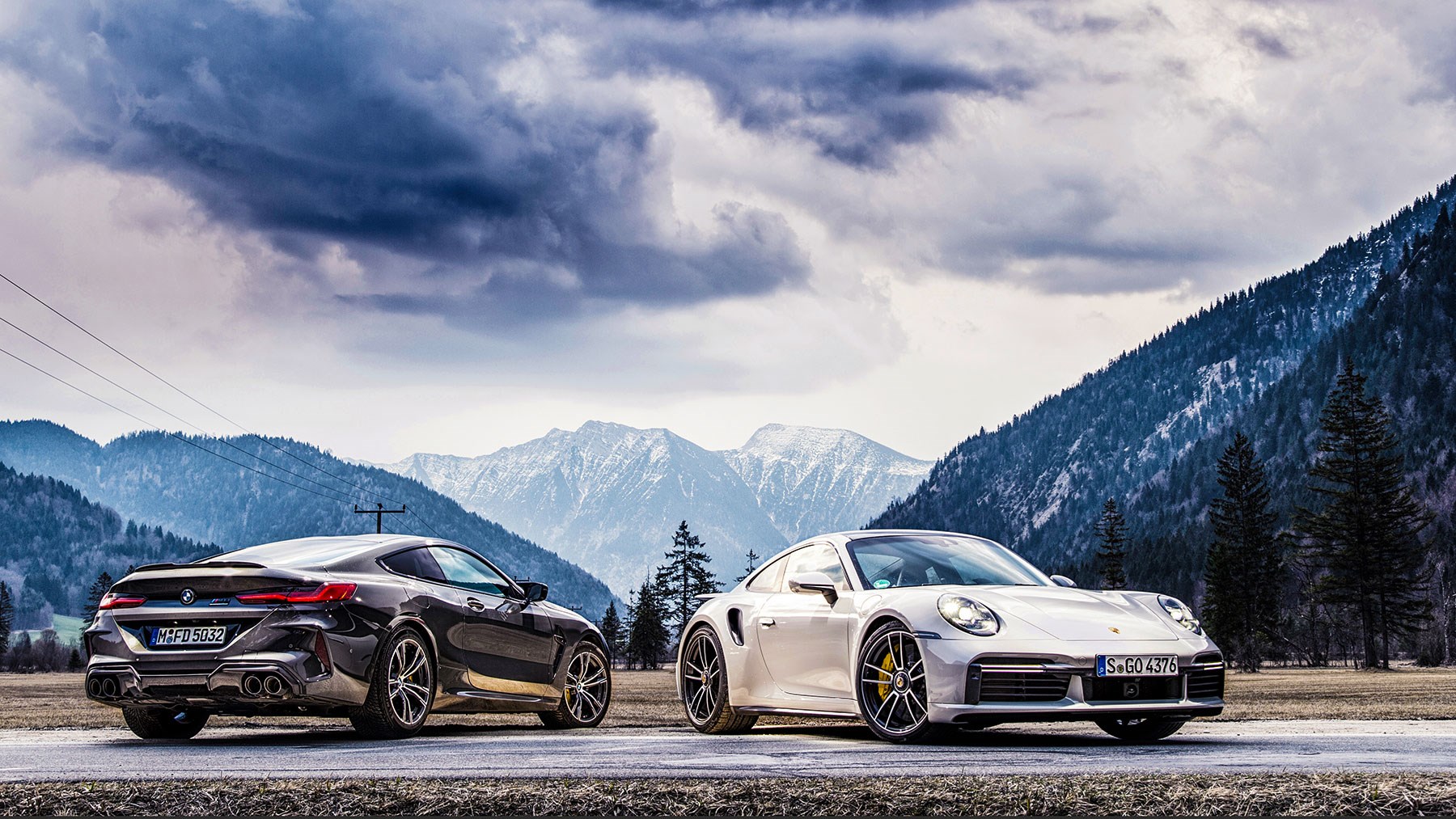In this horizontally aligned rectangular photograph, two sports cars are prominently featured against a dramatic landscape. The image shows a black BMW on the left, identifiable by its logo and the license plate MFD 5032. This sleek, two-door vehicle is parked with its rear visible, highlighting its dual exhaust and red taillights. On the right is a silver Porsche, possibly a 911, with the license plate SG04376. The Porsche is positioned facing forward, allowing a clear view of its distinctive design. Both cars are parked on a narrow paved road, with the edge of the road encroaching into a brown meadow.

In the background, a series of majestic mountains rise into the sky, some capped with patches of snow. Tall pine trees line the left and right sides of the photograph, adding depth to the mountainous backdrop. The sky above is filled with a mix of light and dark gray storm clouds, creating a dramatic and moody atmosphere. Despite the overcast weather, the photograph seems to have an HDR effect, which enhances the vividness and clarity of the car colors and the surrounding landscape. The overall scene is set in a picturesque mountainous area, characterized by a blend of rugged natural beauty and the sleek, modern design of the two featured sports cars.